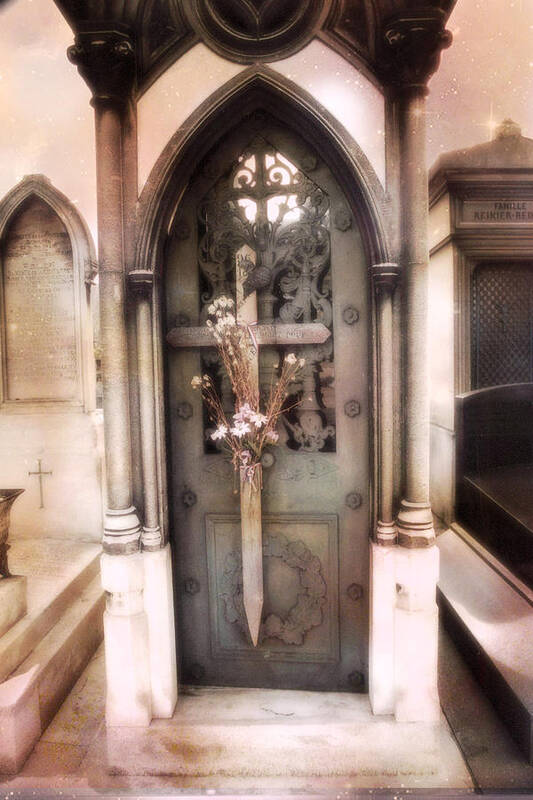The image depicts the front of an ornate tomb or grave, characterized by its gothic architectural style, with a striking mix of black and white detailing. The central focus is a heavy, intricately designed, gray door framed by a small archway. This doorway is adorned with elaborate patterns, including a wreath engraved on the door and flowers lining its edges. Prominently displayed on the door is a large wooden cross adorned with a plant featuring white flowers and green leaves, some of which wrap around the top of the cross. The photograph captures this scene in monochrome, adding to the solemn beauty of the place. On either side of the main tomb are additional tombs; the one on the left has a smaller, imprinted cross at the bottom. The overall ambiance suggests an old-school or gothic aesthetic, highlighted by light shining through the church-like setting.